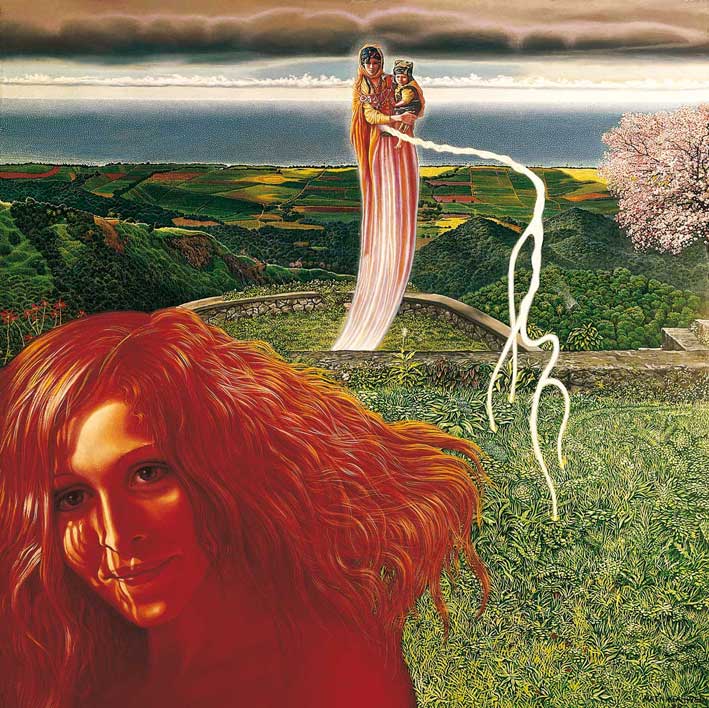The artwork depicted is a detailed, abstract painting featuring vivid characters and a lush, expansive landscape. In the foreground, a deep red-hued woman with wavy hair, her face illuminated by sunlight, dominates the scene. Her skin tone and hair blend seamlessly into the vibrant reds and oranges that define her form. She appears to be in motion, almost as if she's running, with an ethereal quality to her presence. 

Adjacent to her, a tall, slender woman cloaked in a long red and orange gown stands prominently, holding a small child tenderly in her arms. This central figure seems to float above a ledge, her outstretched arm emitting a striking white lightning-like pattern, adding to the fantasy-like atmosphere of the painting.

The background unfolds into a rich, grassy field that transitions into rolling hills and meticulously gridded farmlands. A cherry blossom tree with its soft pink hues stands to the middle left, adding a touch of delicate beauty to the scene. Further in the distance, the landscape extends towards a serene ocean with clouds hovering along the horizon, under a sky that reveals patches of blue allowing beams of sunshine to filter through. The entire scene captures a harmonious blend of natural and fantastical elements, rendering a picturesque, dream-like vision.